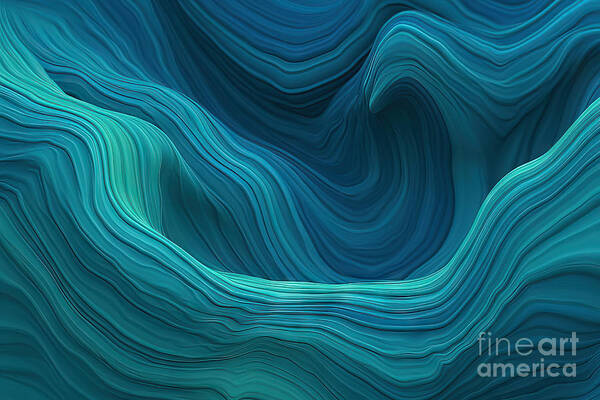This image depicts a computerized abstract artwork featuring wavy, undulating patterns reminiscent of ocean waves or flowing water. The composition predominantly showcases various shades of blue and blue-green, creating a dynamic interplay of colors ranging from light teal to darker blue hues. The design includes high and low wave-like forms that begin in the bottom right corner and cascade in swirling motions across the canvas, culminating in intricate nooks and crevices that give the piece a 3D appearance.

In the foreground, the colors are lighter, transitioning to deeper, darker blues as they recede into the background. A watermark in the lower right-hand corner reads "Fine Art America," with "Fine" in thin print and "Art America" in a bolder font, subtly stamped in a transparent gray. This harmonious blend of flowing lines and gradient colors captures the essence of abstract motion, evoking the serene yet powerful nature of water.